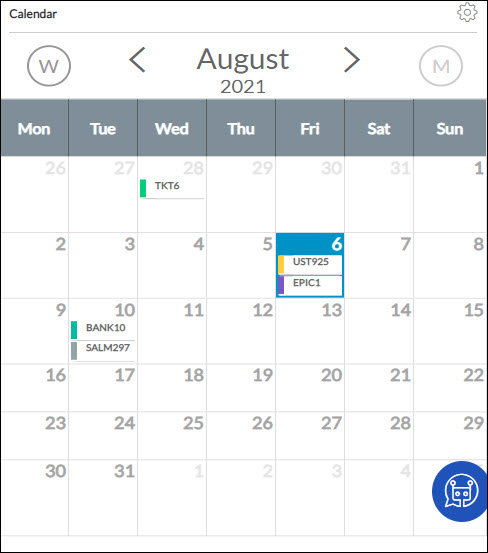The image displays a digital calendar set to August 2021. The overall background is white with "Calendar" written in black letters at the top left of the navigation bar. On the top right of this bar, there is a settings gear icon. Below the navigation bar, there are options to switch between week and month views for August 2021.

The days of the week are displayed in a row with a gray background and white lettering. The calendar starts with Sunday, August 1st, 2021, and ends on Tuesday, August 31st, 2021. There are a total of four complete weeks and two partial weeks, marked by grayed-out sections for the preceding and following months.

Several dates have notes attached to them. On July 28th, a green tag reads "TKT 6." August 6th is highlighted and has two notes: a yellow tag labeled "UST 925" and a purple tag labeled "EPIC 1." August 10th, though not highlighted, features a green tag noting "Bank 10" and a gray tag labeled "SALM 297."